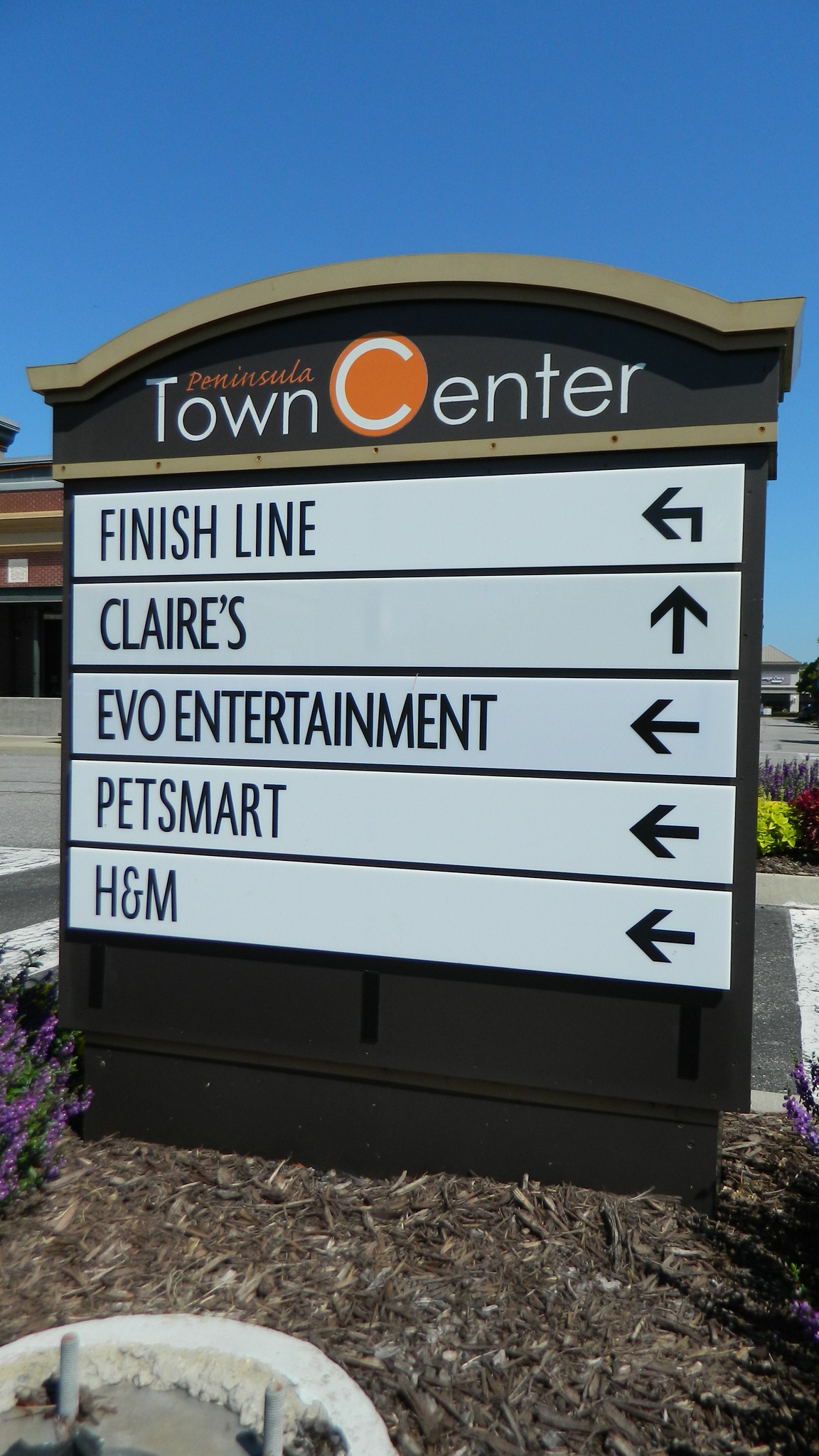This photograph captures the entrance sign to Peninsula Town Center, a bustling plaza. The sign features a prominent gold-topped, rounded design. At its top, "Peninsula Town Center" is prominently displayed, with "C" notably emphasized in white against an orange background, while the rest of the text is white. Below this, smaller text lists several stores housed within the center: Finish Line, Claire's, Evo Entertainment, PetSmart, and H&M. These names are presented in black, all-capital letters on white slatted boards, each with directional arrows indicating their locations. The sign is set in a landscaped median adorned with wood chips. Adjacent to the sign, in the lower left corner, is a section of a white cement structure. In the background, to the left, a storefront is visible, while to the right, the photo reveals part of the plaza's end cap and some colorful flowers. The scene extends to show partial views of the asphalt road on both sides of the sign, under a clear blue sky.